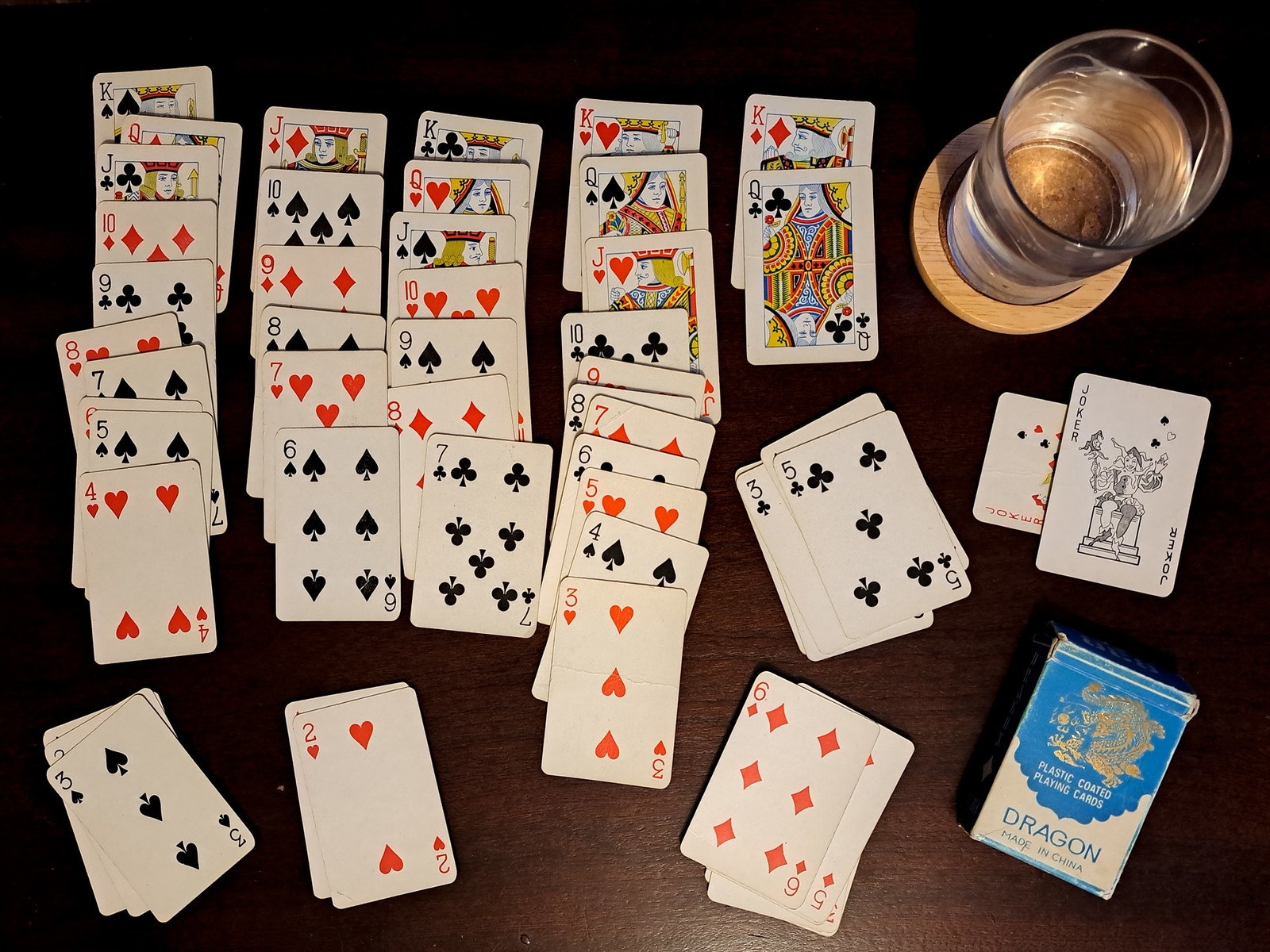The image portrays a rich and dark wooden table surface, on which lies a white and blue pack of playing cards, adorned with a gold dragon graphic and labeled "Dragon, Made in China," situated in the lower right corner. Scattered across the table are various playing cards, arranged haphazardly in columns, representing all four suits: spades, diamonds, hearts, and clubs, along with a joker card. Additionally, a transparent glass cup filled with water rests on a wooden coaster, adding a touch of everyday life to the scene.